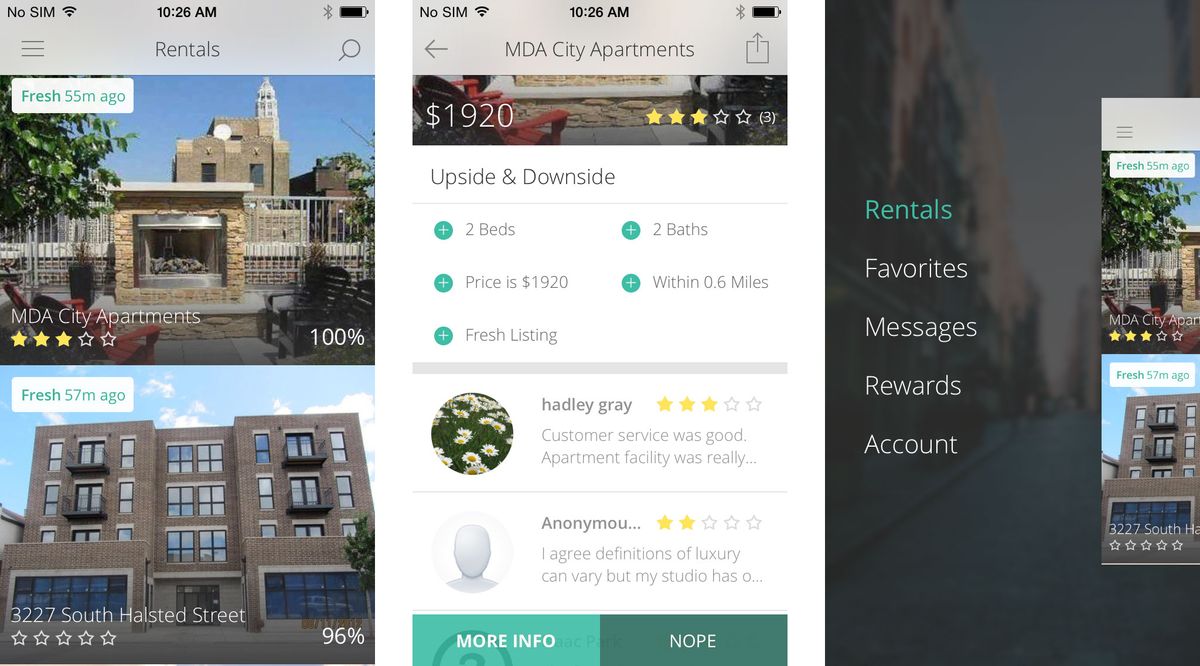The page features three detailed screenshots showcasing different aspects of apartment listings. 

### Screenshot 1:
- **MDA City Apartments:**
  - **Stars:** 3 out of 5
  - **Occupancy:** 100%
  - **Images:** Two pictures of the apartment.
  
- **3227 South Halsted Street:**
  - **Stars:** Not rated yet (stars are blank)
  - **Occupancy:** 96%
  - **Description:** Apartment with numerous windows.

### Screenshot 2:
- **MDA City Apartments Details:**
  - **Size:** Two bedrooms, two baths.
  - **Price:** $1920
  - **Listing Status:** Fresh listing
  - **Distance:** Located within 0.6 miles

- **Reviews:**
  - **Reviewer:** Hadley Gray
    - **Rating:** 3 out of 5 stars
    - **Comment:** "Customer service was really good. Apartment facility was really…" (comment truncated)
  - **Reviewer:** Anonymous
    - **Rating:** 2 out of 5 stars
    - **Comment:** "I agree definitions of luxuries can vary but my studio has…" (comment truncated)

### Screenshot 3:
- **Additional Options:**
  - **Buttons:** 'More Info' and 'Nope' (in green)

This descriptive review offers a comprehensive look at the two apartment listings, detailing ratings, occupancy, and reviews, giving potential renters a clear snapshot of their options.